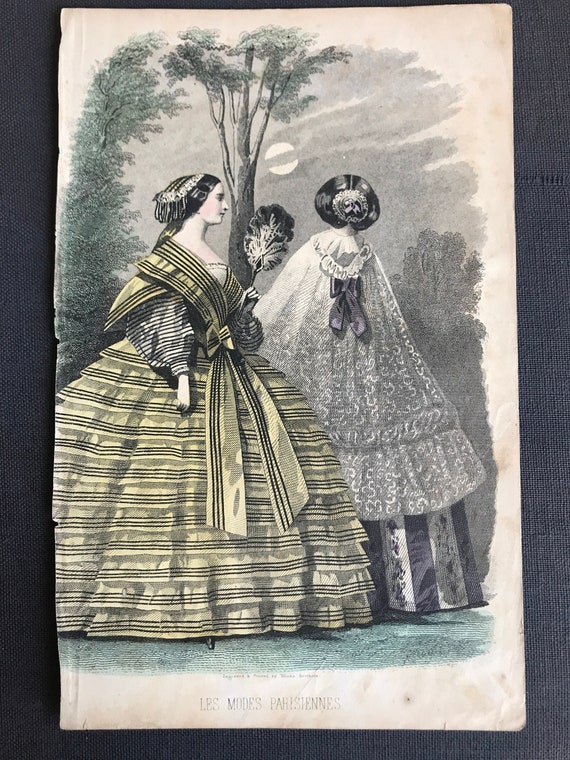This is a detailed color illustration that resembles an old text, with the edges of the page yellowed and slightly torn. The artwork, labeled in French as "Les Modes Parisiennes," which translates to "Parisian Fashions," shows two women dressed in extravagant, bell-shaped dresses indicative of the 1700s or 1800s. The woman in the foreground to the left is adorned in a yellow dress with horizontal black stripes and multiple layered ruffles, numbering twelve, each wider than the previous. She gazes to the right and has elaborate hair accessories, including a white cloth with dangling strings. The woman to the right is depicted from the back, wearing a lacy top that extends almost to the ground, over a vertically-striped dark blue and white dress. The painting is affixed on a black cloth surface, embodying an antique aesthetic with its brown-shaded, coarse-edged paper.